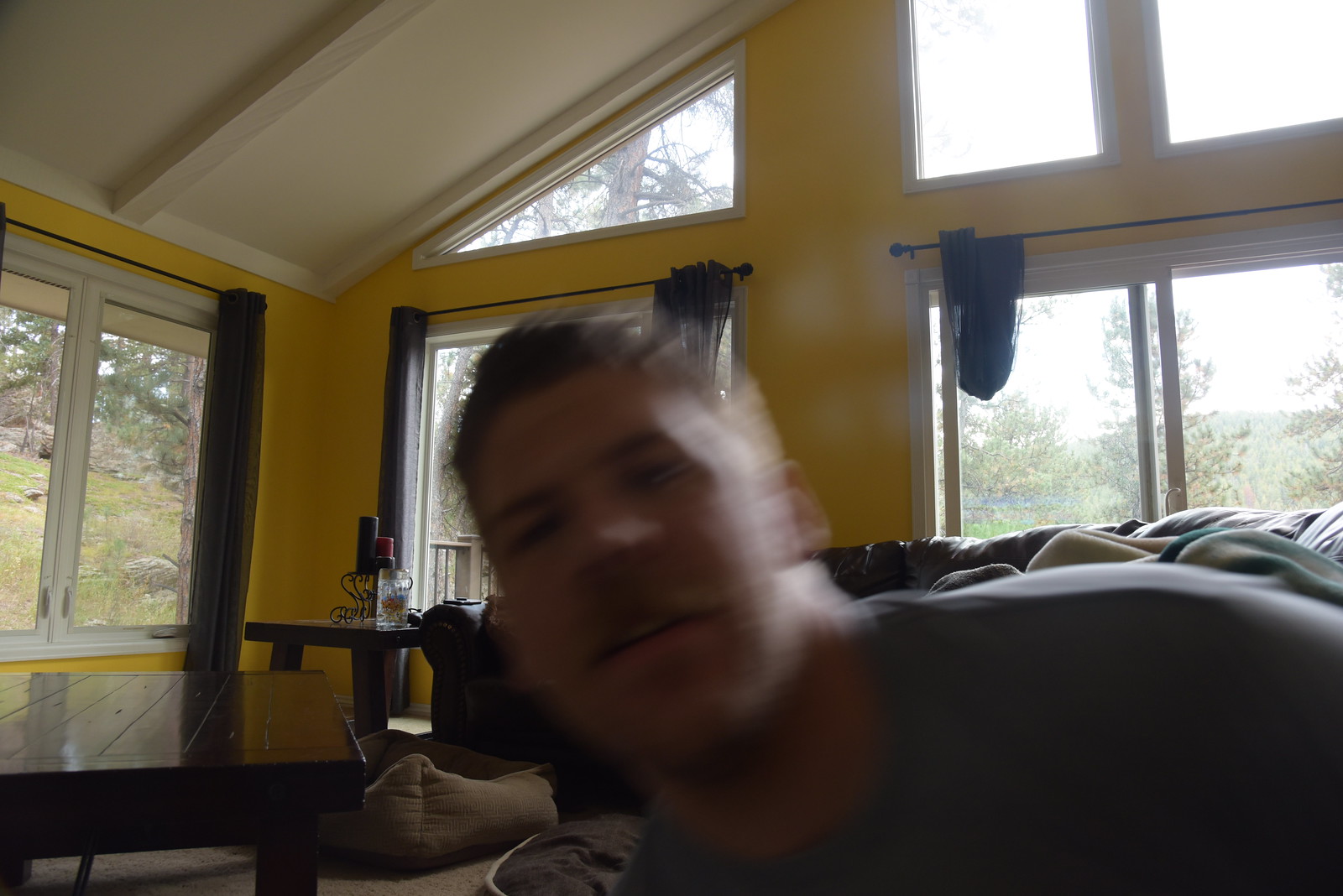In the image, a young to middle-aged Caucasian man, possibly in his 30s, with short, light brown or dark blonde hair that appears slicked back, stands blurry and out of focus in the foreground. He is wearing a gray short-sleeved t-shirt and sporting a mustache. The man's head is tilted toward the top left corner of the image, as if he's leaning to get into the center of the shot, creating an extremely blurry presence.

The background is in sharp contrast, being very clear and showcasing a spacious, modern room with a vaulted, A-frame ceiling accentuated by white paneling and beams. The room is bathed in natural light streaming through numerous large, floor-to-ceiling height windows and sliding glass doors, some of which have curtains looped up to the side. The walls are painted a vibrant buttery yellow with dark wooden trim adding a touch of warmth. Further adding to the modern aesthetic, the ceiling in some parts appears tan.

Prominent in the background are natural, wooded surroundings visible through the expansive windows, which reveal a scenic landscape of trees, hills, and boulders. Inside the room, dark wooden furniture pieces are evident, including two tables on the left-hand side, one adorned with a glass jar and an ornate cast-iron pillar candle holder. There is also a mention of dark furniture like leather couches, perhaps a bed, and possibly some bean bags, reflecting a well-furnished, open, and airy living space.